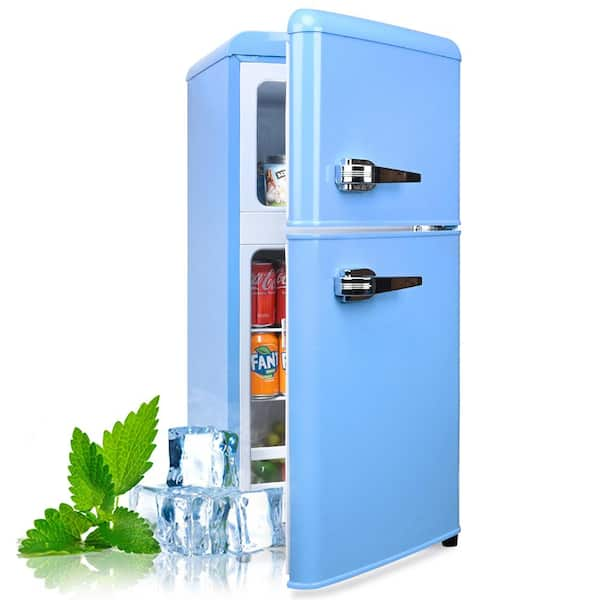The photograph features a retro-style, baby blue mini-fridge with silver handles. The fridge has its door ajar, revealing three shelves inside. The lower two shelves contain 12-ounce cans of soda, with the top shelf located below a small freezer compartment that holds a carton of ice cream. The size of the fridge is small, evidenced by the fact that each shelf can only accommodate a single can's height, suggesting a compact design suitable for small spaces like hotel rooms or college dorms. Outside and to the left of the fridge, there are several large ice cubes stacked with a sprig of mint, possibly symbolizing freshness. The legible soda brand in the image is Orange Fanta, adding a splash of color and detail to the overall scene.